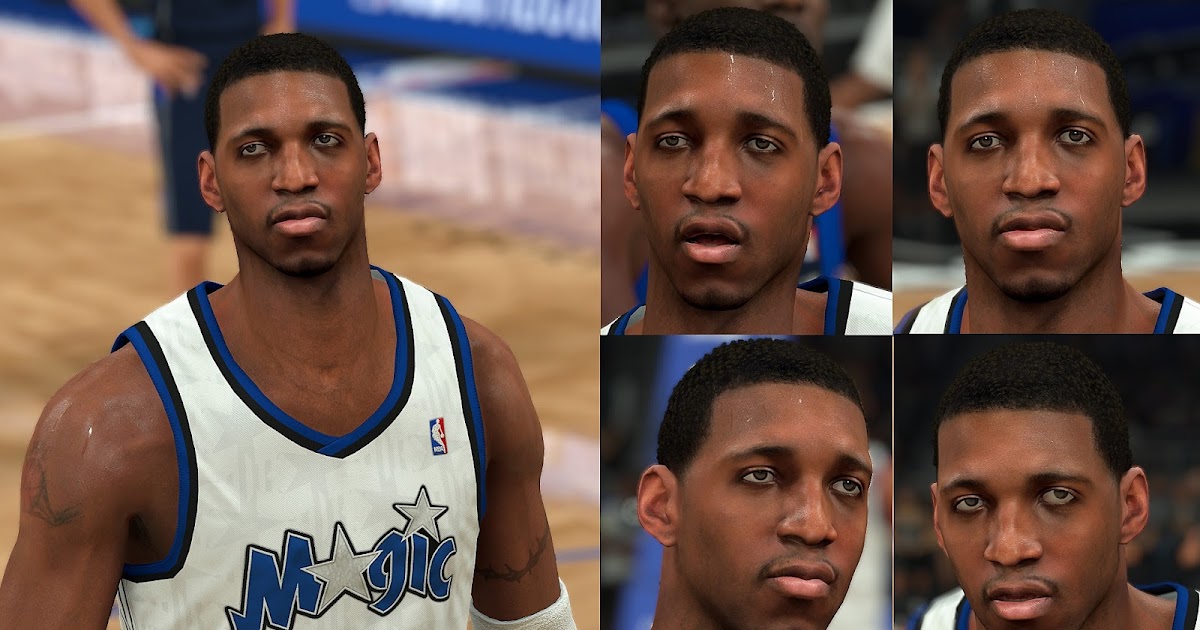This series of images showcases NBA legend Tracy McGrady, likely sourced from an NBA 2K video game. The images capture McGrady during his early career with the Orlando Magic. Four square boxes aligned on the right highlight close-ups of his face, each portraying different expressions. These virtual renderings are impressively realistic, right down to the sweat glistening on his face and his subtle mustache.

On the left, a single box presents McGrady standing on the basketball court in his iconic Magic uniform. The white jersey features the word "Magic" in blue, with star motifs replacing the 'A' and the dots in 'I.' The uniform is detailed with blue and black accents along the collar and shoulders. McGrady, with his dark complexion, is also seen sporting a white elbow pad.

The background, although blurry, hints at the atmosphere of a live basketball game, drawing all focus towards McGrady. Known for his extraordinary skills, Tracy McGrady is widely celebrated as one of the best basketball players of all time and a Hall of Famer who dominated the sport in the early to mid-2000s.